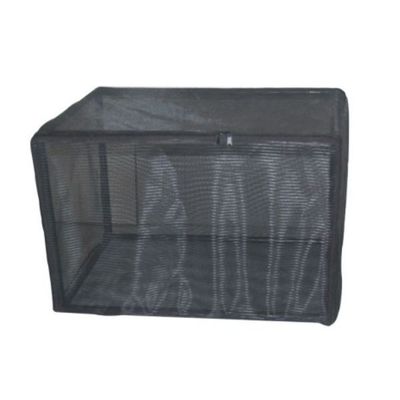The image depicts a rectangular, black mesh storage item, possibly a pet kennel or a laundry hamper, set against a plain white background. This three-dimensional box features a metal frame overlaid with a semi-transparent mesh material, allowing visibility through all sides. The box has a couple of zippers on the upper edge at the front, suggesting it can open from the top. While the corners of the structure are solid, the rest of the item is notably made of mesh, providing a lightweight and airy design. There may be another rectangular feature inside or on the far side of the box, hinting at additional compartments or a door. The absence of any logos or objects for scale leaves the precise size undetermined.